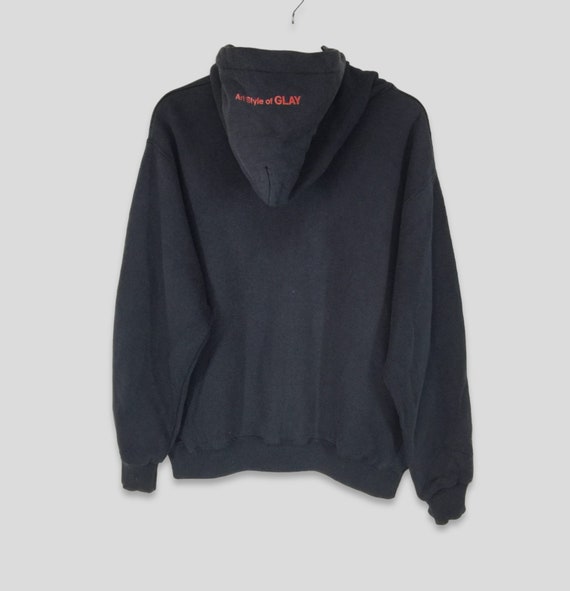In this close-up, portrait-oriented photograph, a suspended, black hoodie takes center stage against a high-contrast white and gray backdrop. The hoodie is hung on what appears to be a transparent hanger, with only a small silver hook visible at the top of the image. The garment itself is slightly faded and features large, oversized sleeves with cuffs at the wrists and waist. The hoodie is displayed from the back, showing a hood that drapes down and prominently displays the text "Art Style of GLEI." The text is in a vibrant red or orange hue, with "Art Style of" in lowercase letters and "GLEI" in a larger, uppercase font, emphasizing the latter.